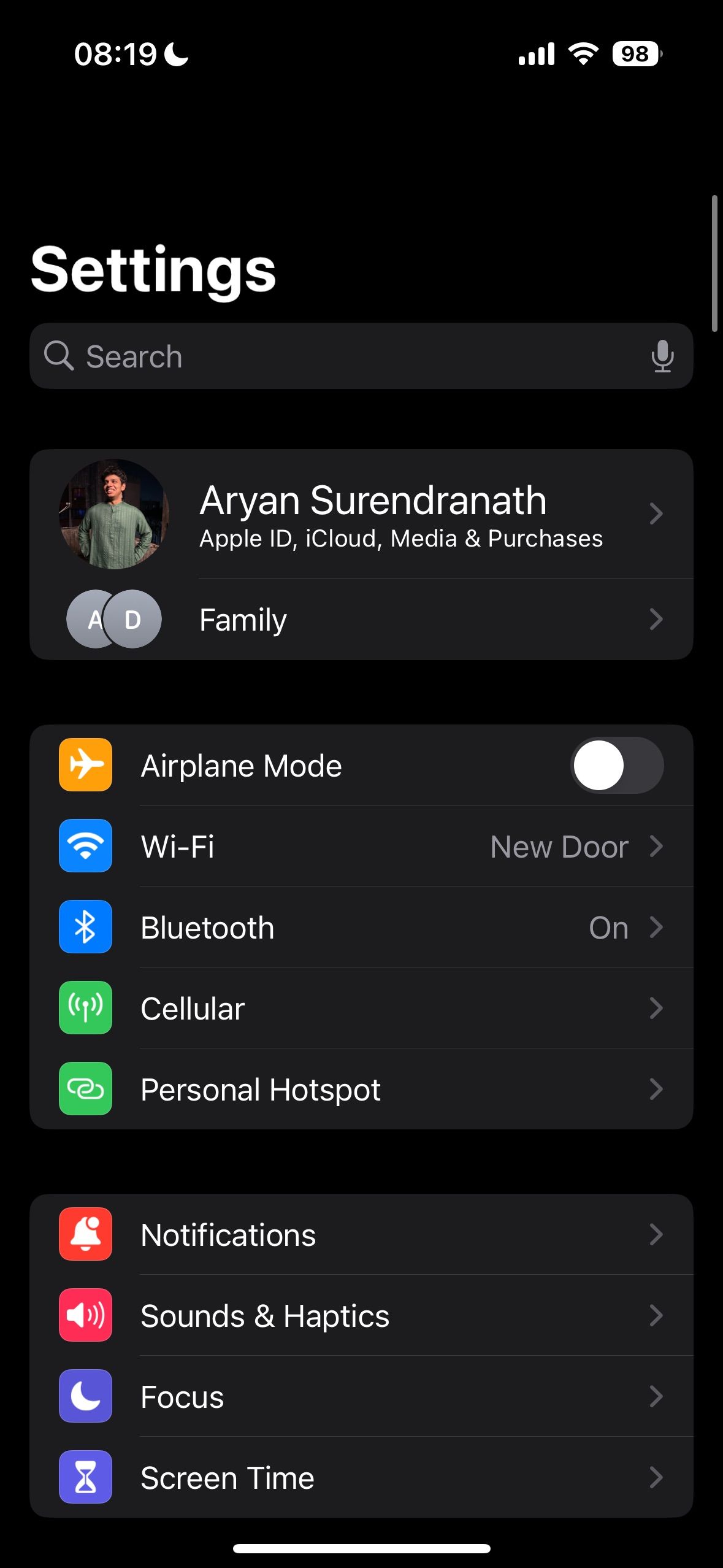A detailed screenshot of a smartphone's top section, oriented sideways, set against a black background. The status bar at the top displays "0819" in white, with a moon icon beside it, indicating it is 8:19 PM. On the right-hand side of the status bar, a series of four ascending bars depict the cellular signal strength, alongside a Wi-Fi symbol and a battery icon showing 98% charge.

Directly below the status bar is the word "Settings" in white, followed by a search bar featuring a magnifying glass icon on the left and a microphone icon on the right. Beneath this search bar is a profile section displaying a picture of an individual in a green shirt. Further down, a circular icon contains the letter "A," slightly overlapped by another circle with the letter "D". The text "ARYAN SURENDRANATH" follows, with additional descriptors "Apple ID, iCloud, Media and Purchases, Family."

The screenshot continues to display various phone modes: "Airplane Mode," "Wi-Fi," "Bluetooth," "Cellular," and "Personal Hotspot," each accompanied by their respective icons. A black spacer bar separates these from another set of icons below, which includes "Notifications," "Sounds & Haptics," "Focus," and "Screen Time."